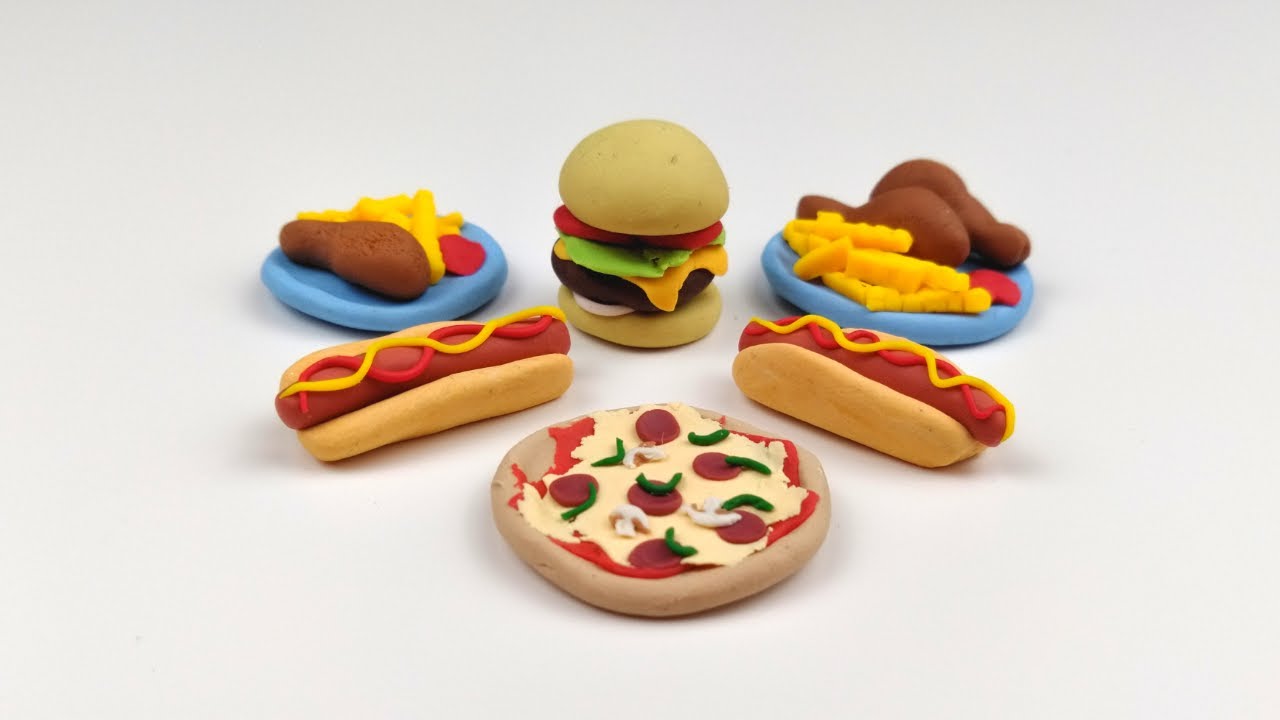The photograph showcases an array of meticulously sculpted food items made entirely out of colorful Play-Doh, displayed on a pristine white surface. Central to the display is a blue Play-Doh plate holding vibrant yellow Play-Doh fries, two brown Play-Doh chicken legs, and a small red Play-Doh blob mimicking ketchup. Adjacent to the plate lies a cream-colored Play-Doh disc decorated with shredded red Play-Doh to imitate pizza sauce, topped with small red discs representing pepperoni slices. Nearby, a Play-Doh hot dog is crafted with a bun, sausage, and condiments. Completing the display is a Play-Doh hamburger, detailed with distinguishable layers: a red slice of tomato, a green piece of lettuce, a yellow cheese slice, and a brown patty, all nestled within a bun. The intricate details and vivid colors bring a playful and creative culinary scene to life.